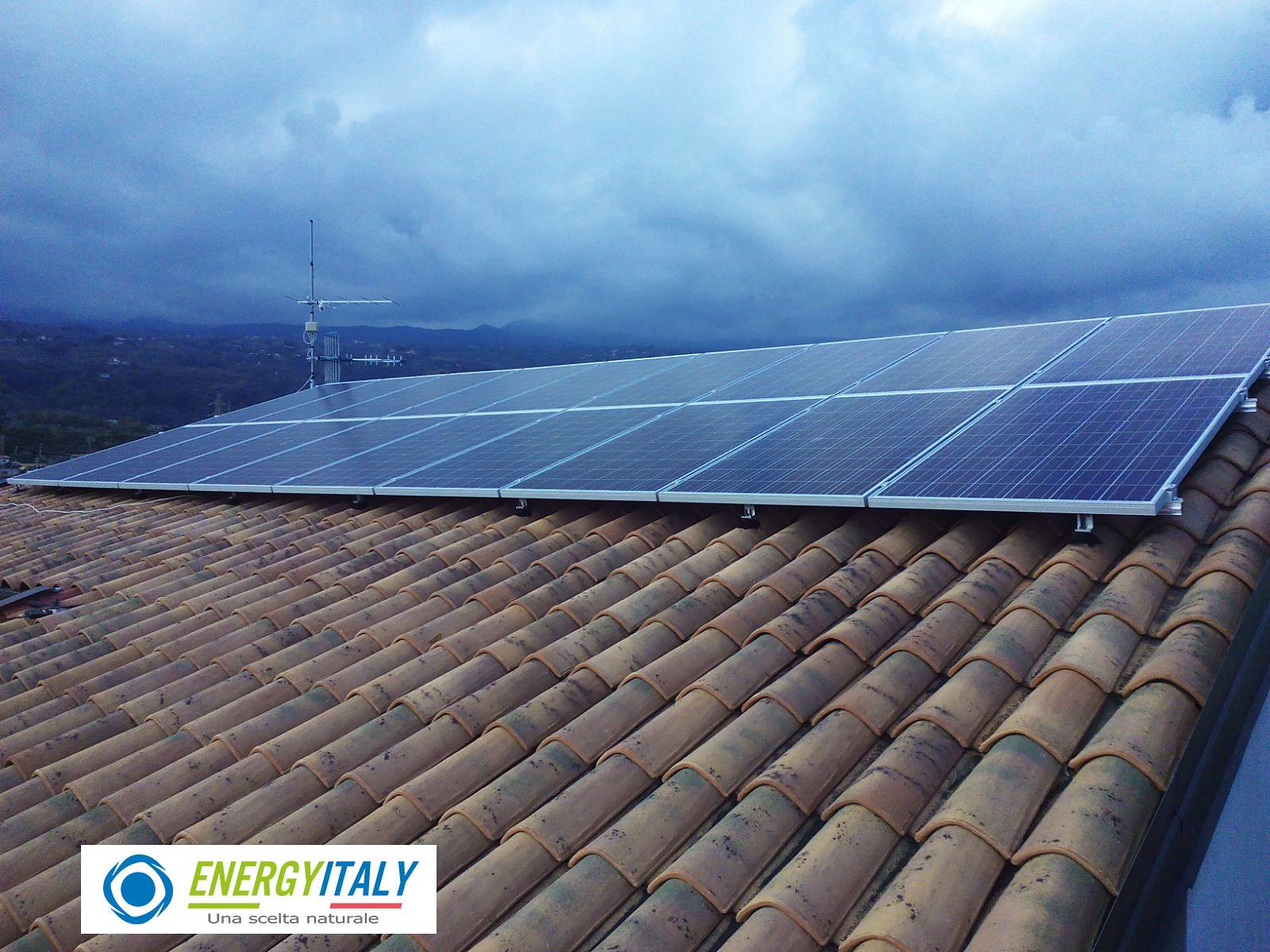The photograph captures a roof with aged, terracotta shingles; the tiles are faded and blackened in some areas. The roof is adorned with 18 rectangular solar panels extending from one side to the other, clipped in place with silver fasteners. Toward the end of the roof, an antenna-like structure is visible. The backdrop features a dramatic skyline with dark, stormy clouds and distant hills, providing a contrasting natural element. In the lower left corner of the image, a white box displays the logo "ENERGY ITALY" with distinct color details: "ENERGY" in green, "ITALY" in blue, underlined by green and red lines, respectively. Below the text reads, "UNA SCELTA NATURAL." The logo is accompanied by a blue circle and a diamond shape, completing the visual narrative of sustainable energy amidst a moody, cloud-laden landscape.